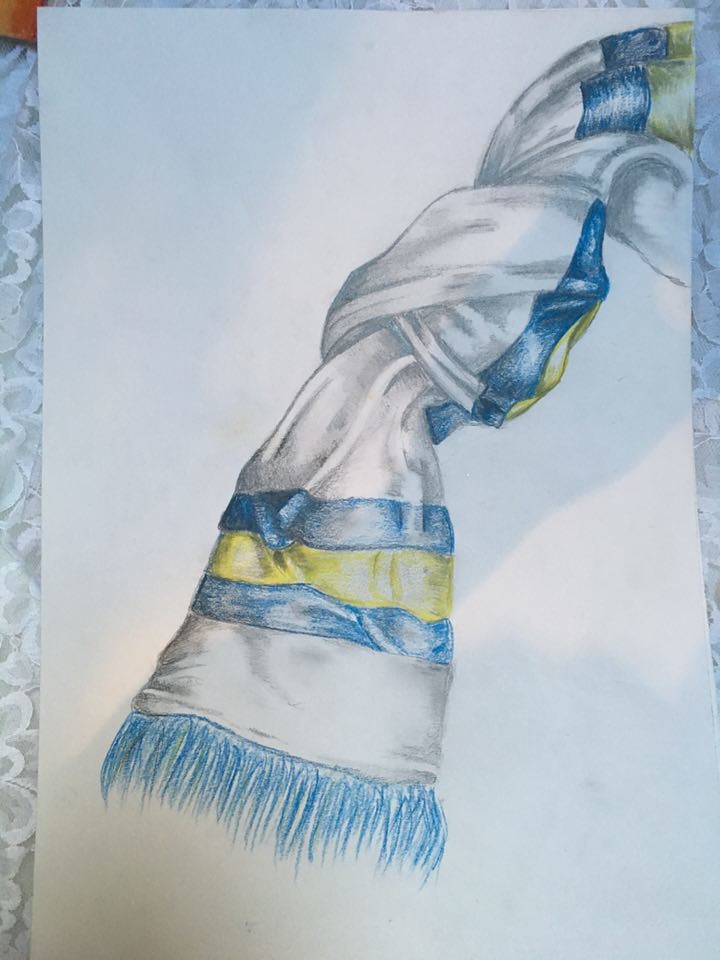The image features a hand-drawn scarf on a white piece of paper, positioned vertically atop what appears to be a lace tablecloth or a lace curtain. The drawing, possibly rendered in colored charcoal, depicts a primarily white scarf adorned with three sections of stripes. These sections are located toward the left, right, and center of the scarf. Each section consists of a medium blue stripe, a yellow stripe, and another medium blue stripe. The knot of the scarf is situated slightly above the center of the image. Additionally, blue fringe is visible hanging down from the forefront of the scarf, though the fringe on the right side extends beyond the edge of the paper and is not visible. The detailed composition highlights the striped pattern and subtle positioning nuances in the scarf’s design.